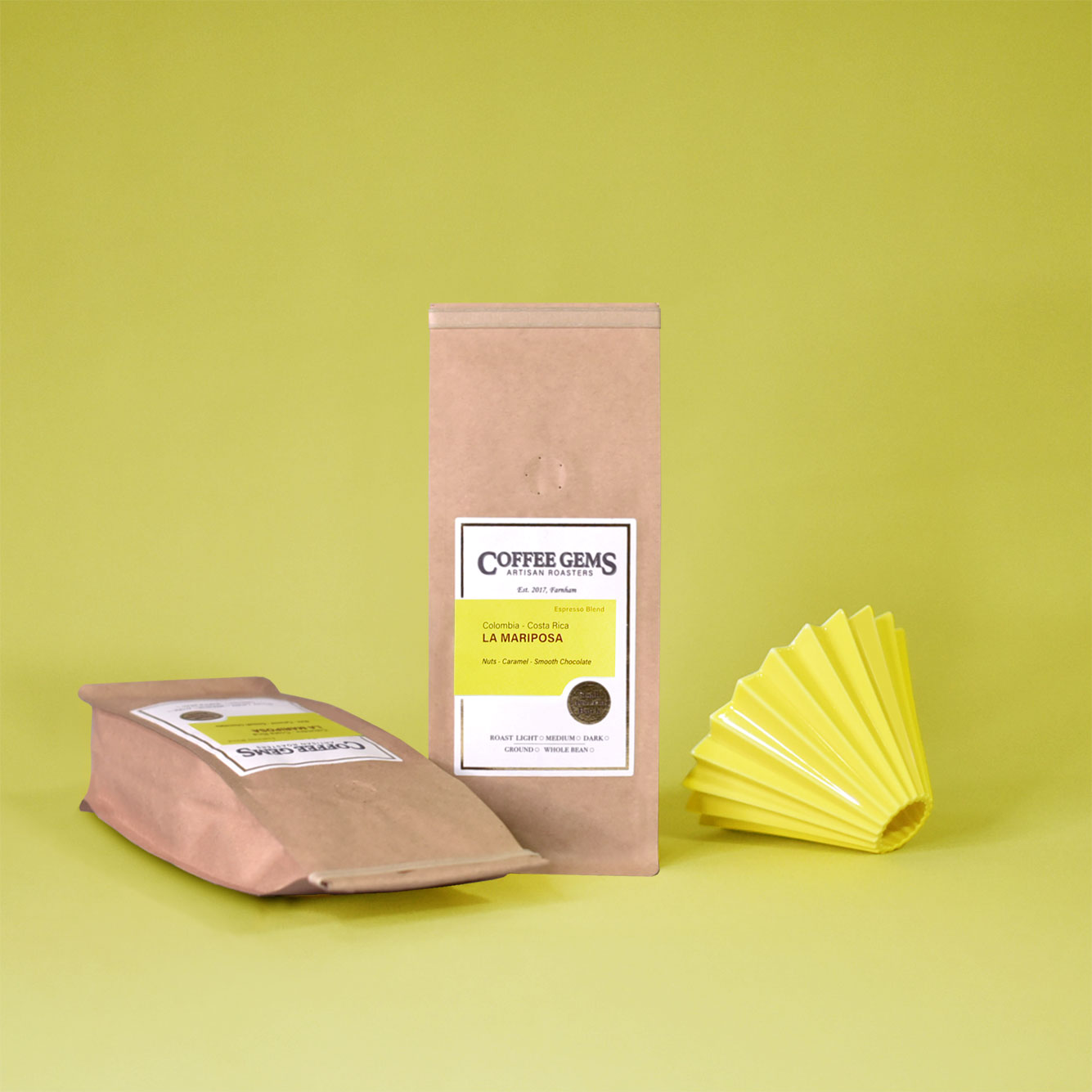This image features two brown paper bags of gourmet coffee against a lime to chartreuse green gradient background that darkens towards the top. The bags are labeled "Coffee Gems" and "Artisan Roasters," with a prominent white label edged in black. The label features the coffee name "La Mariposa" in a yellow rectangle. The taste profile is noted as having flavors of nuts, caramel, smooth chocolate, and the coffee is available in various roast levels and ground forms. One bag stands upright, while the other lies on its side, showcasing the label. To the right, an intriguing cone-shaped object with wavy patterns resembling a decorative paper fan adds a unique visual element.